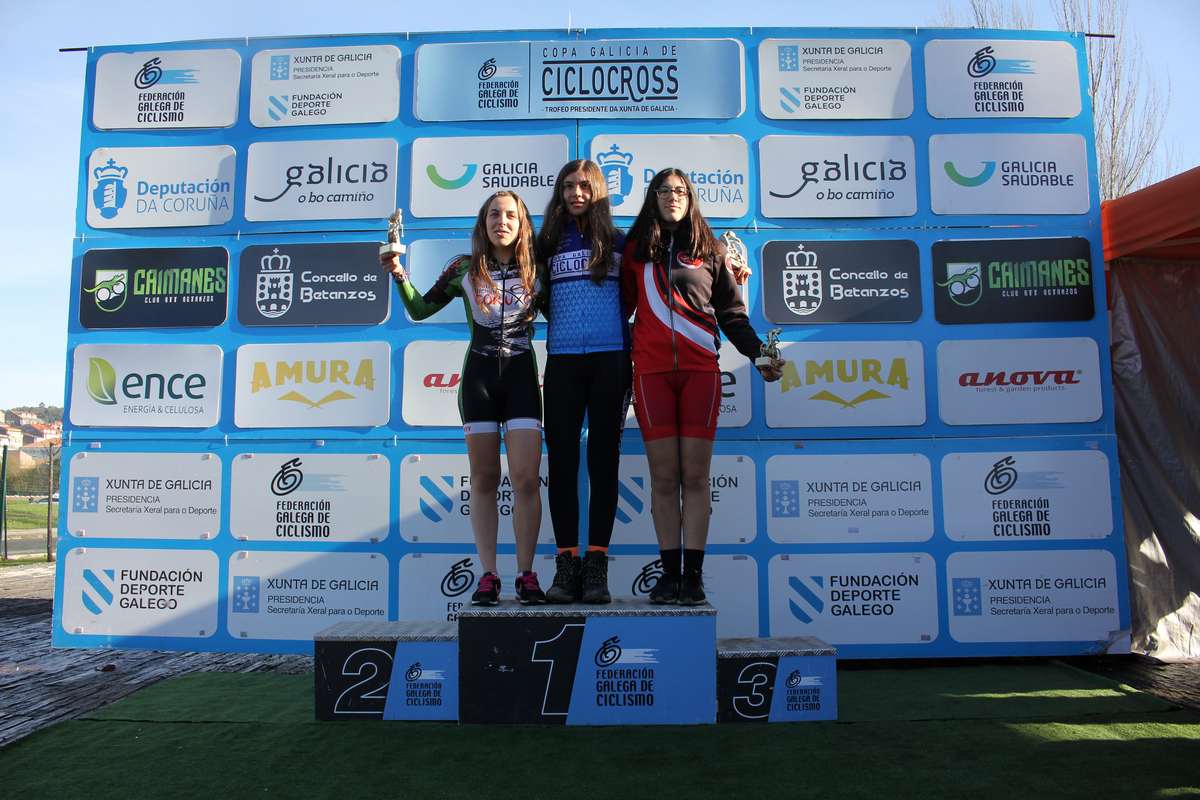In this photograph, three sports players are proudly standing on the top tier of a three-tier podium situated in an outdoor venue. Each player has a trophy in hand, signifying their achievement, and they have draped their arms around each other's shoulders and backs, showcasing camaraderie and team spirit. Curiously, the second and third tiers of the podium are conspicuously vacant, directing all attention to the top. The podium itself is covered in a green-colored sheet, adding a vibrant touch to the scene. Behind the athletes is an expansive banner adorned with an array of logos and names from various sponsoring companies. Above this banner, a clear blue sky stretches out, providing a picturesque backdrop to the triumphant moment.